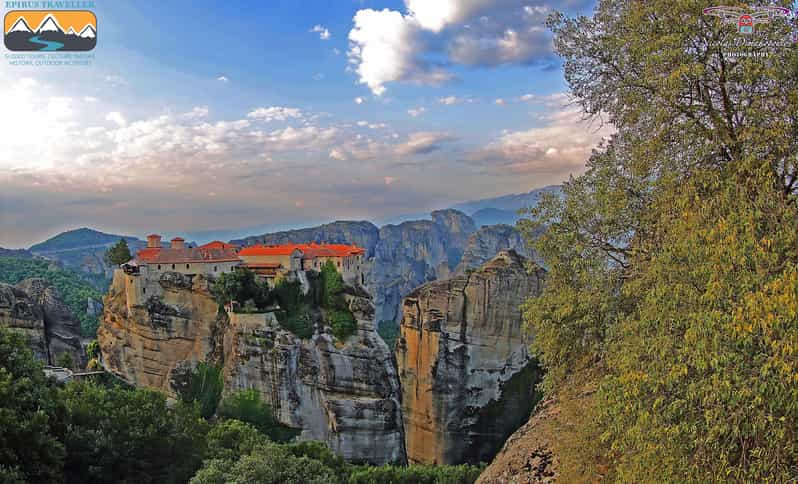The image is a detailed painting of a scenic mountain landscape. In the foreground on the right side, a large tree with green leaves and brown branches occupies about a quarter of the image. The tree is not the focal point, as attention is drawn to the center of the composition. Here, a long, one or two-story building with an orange roof is precariously perched on a narrow, rocky ridge, giving the appearance of a villa in an isolated mountaintop setting. The rocky ridge and the mountainous background feature hues of gray, black, and brown, with additional greenery scattered around.

Beyond the ridge, a majestic range of rugged, rocky mountains stretches across the horizon, appearing untouched and naturally beautiful. The sky above is a vibrant blue adorned with white clouds, and as it descends, it transitions into a subtle pinkish hue near the horizon, enhancing the dramatic and serene atmosphere of the scene. Surrounding the mountains and the central building are multiple trees, varying in shades of green, contributing to the lush and vibrant landscape.

In the upper left corner of the image, there is a logo for "Epirus Traveler," depicted as a rectangle with an orange top, white mountain ranges, black trees, and a blue road. The text "Epirus Traveler" is inscribed in blue. This detailed depiction captures the essence of a tranquil, elevated retreat amidst breathtaking natural beauty.